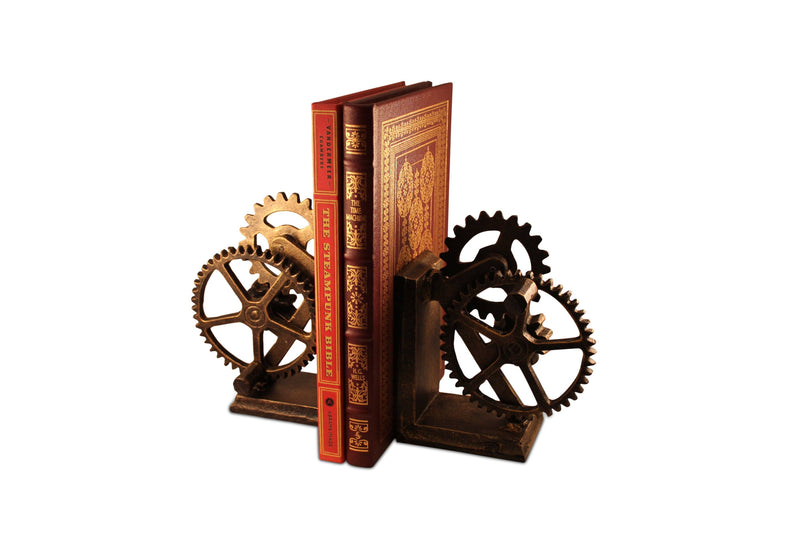The image depicts a creative and intricate steampunk-themed bookshelf against a white background. The focal point includes two hardbound books supported by unique bookends. The book on the left is red with gold lettering on the spine that reads "The Steampunk Bible." The book on the right, titled "The Time Machine," has a dark brown cover adorned with ornate filigree and an intricate gold design. The innovative bookends are in the form of L-shaped brackets, made of dark, bevelled-looking wood and are adorned with two large metallic gears each—one big and one small—secured to the vertical and horizontal parts of the wood, creating a mechanical, steampunk aesthetic. This setup not only secures the books upright but also allows for additional books to be added, maintaining both functionality and visual appeal. The overall design exudes a fancy, vintage charm that is both creative and innovative.